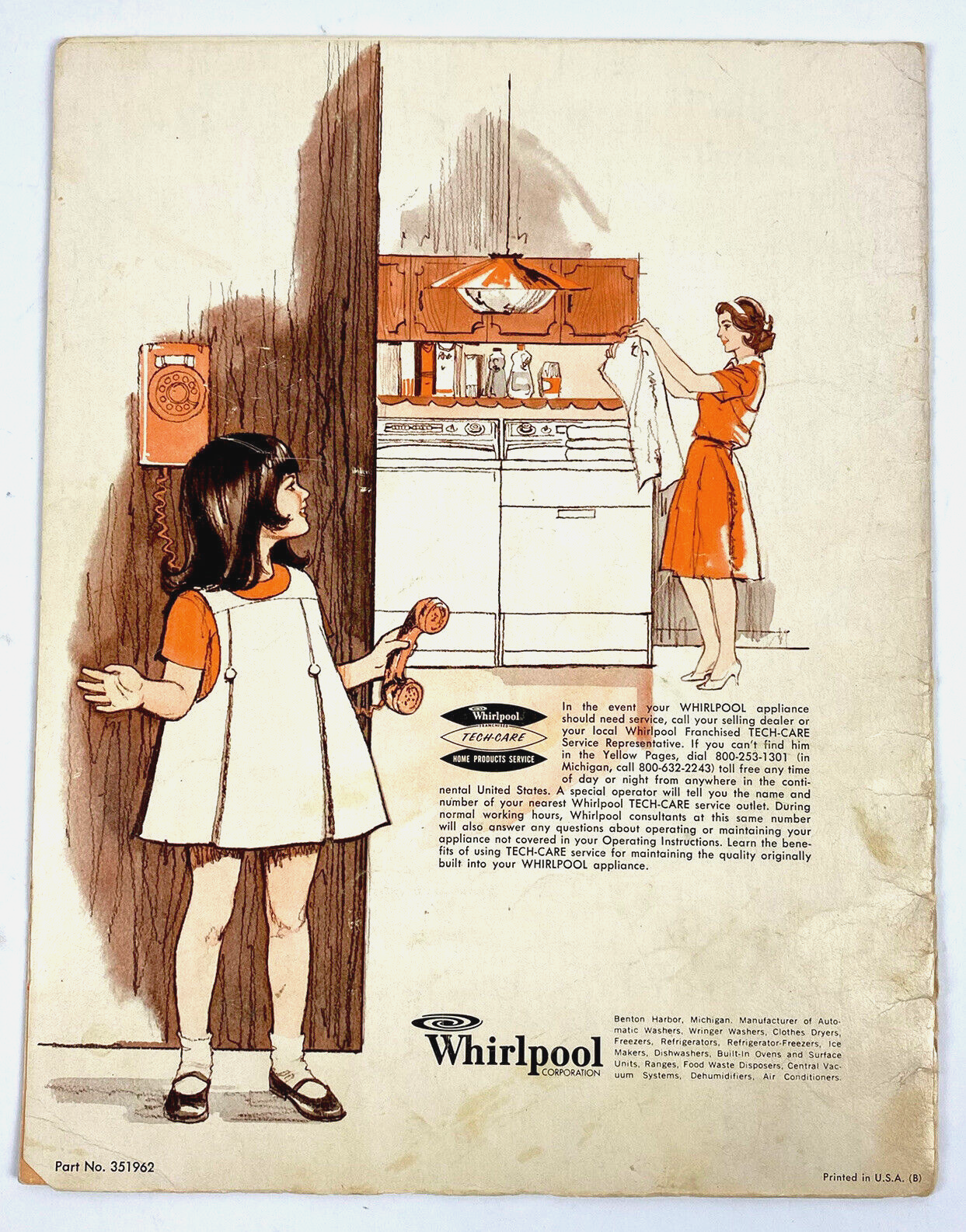This full-page Whirlpool advertisement, seemingly from a vintage magazine, features a domestic scene emblematic of the late 1950s or early 1960s. The focal point is a little girl dressed in a short white jumper over an orange short-sleeved shirt, paired with black shoes and white cuffed socks. She stands against a wood-paneled wall, holding the receiver of a corded wall-mounted telephone, peering around the corner at her mother. In the background, the mother is depicted beside a white washer-dryer combo, dressed in an orange dress and high-heeled shoes, examining a piece of white clothing she’s holding up. At the bottom of the ad, below the mother, is a block of text, alongside the prominently displayed Whirlpool logo. This nostalgic portrayal underscores the fashion and domestic ideals of the era, emphasizing the woman engaged in household chores while dressed impeccably.